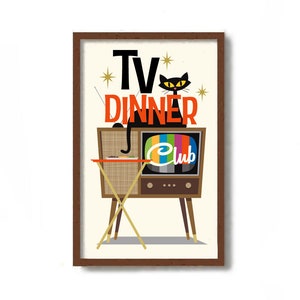This image is a framed print with a brown outline and a vintage 1950s aesthetic. The piece is titled "TV Dinner Club," indicated by the text inside the frame: "TV" in black at the top, "dinner" in red below it, and "club" in white displayed on the screen of an old-fashioned analog television. The TV, which has a thick, heavy build with knobs and a side speaker, is showing a color calibration test pattern with vertical stripes in green, yellow, blue, purple, and red. Perched atop the TV is a black cat with yellow eyes and a notably thin neck. The background incorporates star decorations around the word "TV." Adding to the retro feel, there's a small TV tray table with gold legs and a red top situated in front of the TV. The print is set against a yellowish piece of paper, emphasizing its graphic design roots.